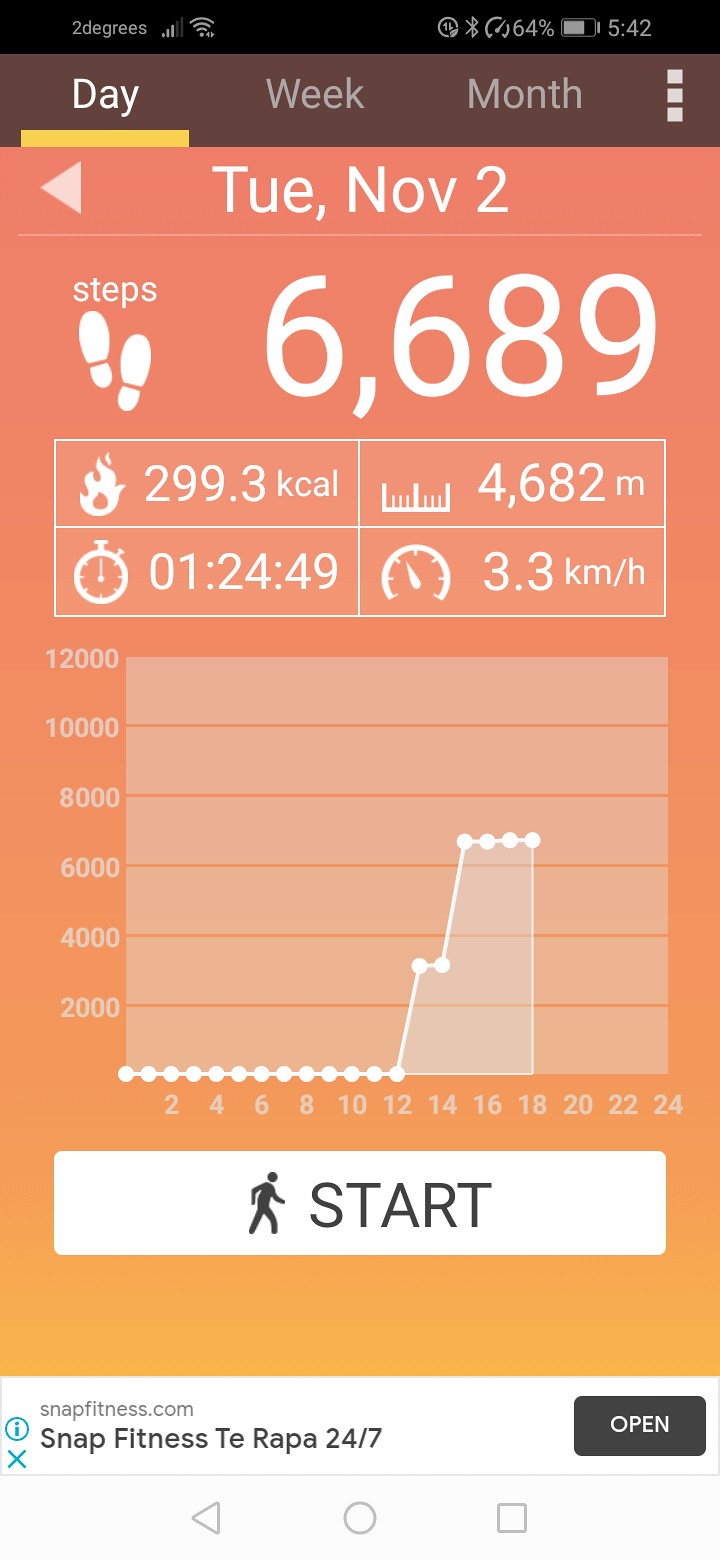The image is a screenshot from a smartphone displaying a fitness tracking app. At the top of the screen, there is a status bar showing cellular signal, Wi-Fi signal, Bluetooth connection, 64% battery level, and the time, 5:42. The topmost section of the app interface features a dark brown banner with the options "Day," "Week," and "Month," with "Day" being highlighted and underlined in yellow. Below this, the date is displayed as Tuesday, November 2nd. There's a large, prominent step count showing 6,689 steps with the word "steps" above it, accompanied by a footprint icon. Further, it lists additional data: 299.3 kcal with a fire symbol, 4,682 meters with a ruler icon, a timer showing 01:24:49, and a speedometer indicating a pace of 3.3 km/h. Below these metrics, there is a line graph that maps steps taken throughout the day, with vertical numbers ranging from 2,000 to 12,000 and horizontal numbers from 2 to 24, suggesting hourly intervals. At the bottom of the screen, there's a large white button with a black silhouette of a man and the word "Start." The background of the app features an orange to yellow gradient.